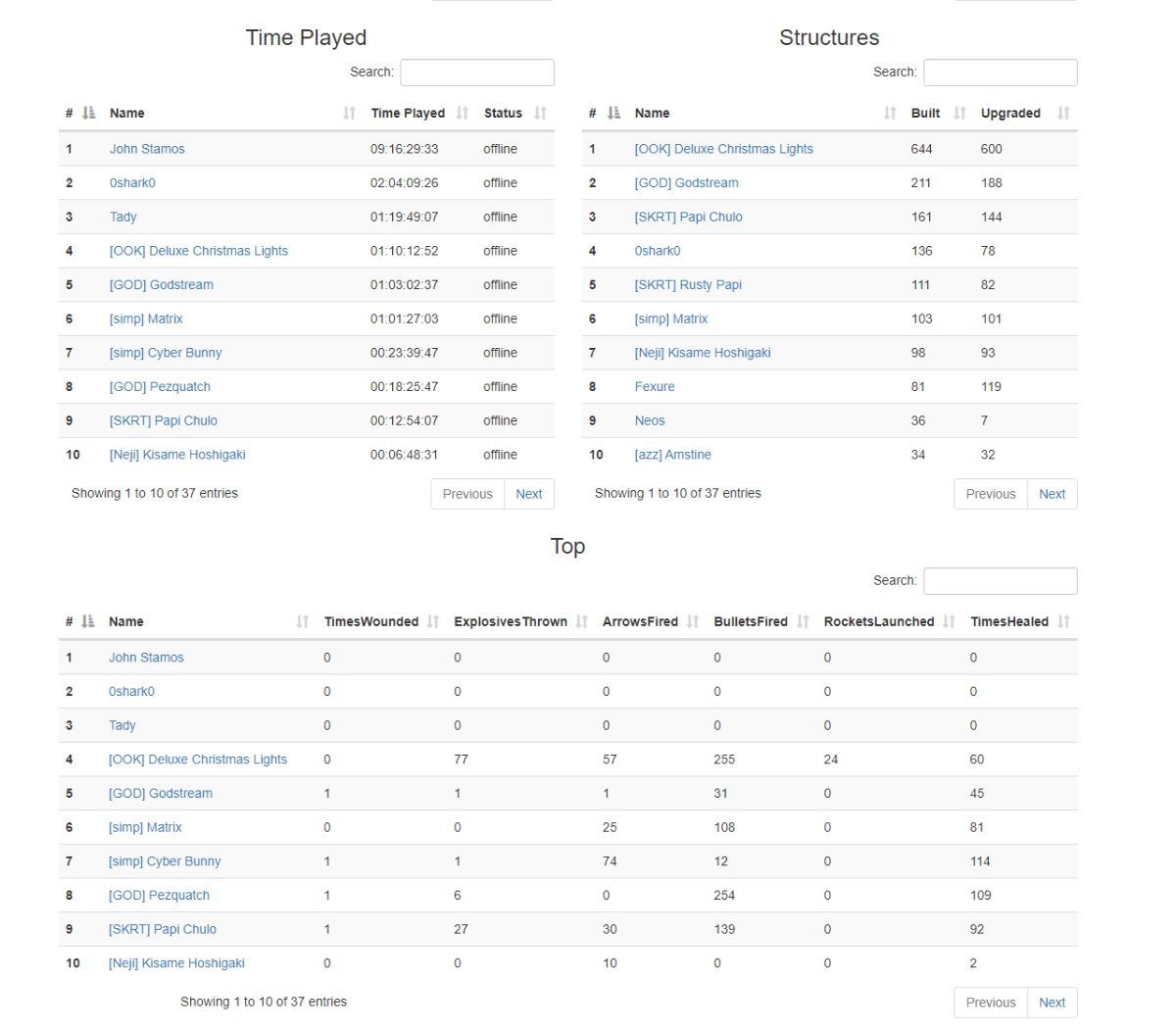In this image, there are two primary columns of information. The first column, labeled "Time Played," and the second column, labeled "Structures," both feature titles in black text. Above these headings, there is a gray horizontal line extending to the top right of the image. Beneath each of these headings, a search box is positioned in the right part of the column, outlined in gray. 

Both columns contain several rows of information, where each row includes blue text accompanied by a black number positioned to its left. For the "Time Played" column, the status of all entries is marked as "Offline," displayed in black text. In the "Structures" column, each entry includes a blue text label, a corresponding number in black, and additional details indicating the quantity built and upgraded. The columns also feature arrows that allow sorting the entries in ascending or descending order.

At the bottom of the columns, navigation buttons labeled "Previous" and "Next" are present. These buttons are outlined in gray with a white background, where "Next" is highlighted in blue text, and "Previous" is in gray text. 

A large section of rows, equivalent in size to the combined height of the two columns, appears below these elements. This section is marked with a heading in black text that reads "Top" and mirrors the layout and features of the upper columns, including the rows of blue text accompanied by black numbers, the sorting arrows, and the search box.